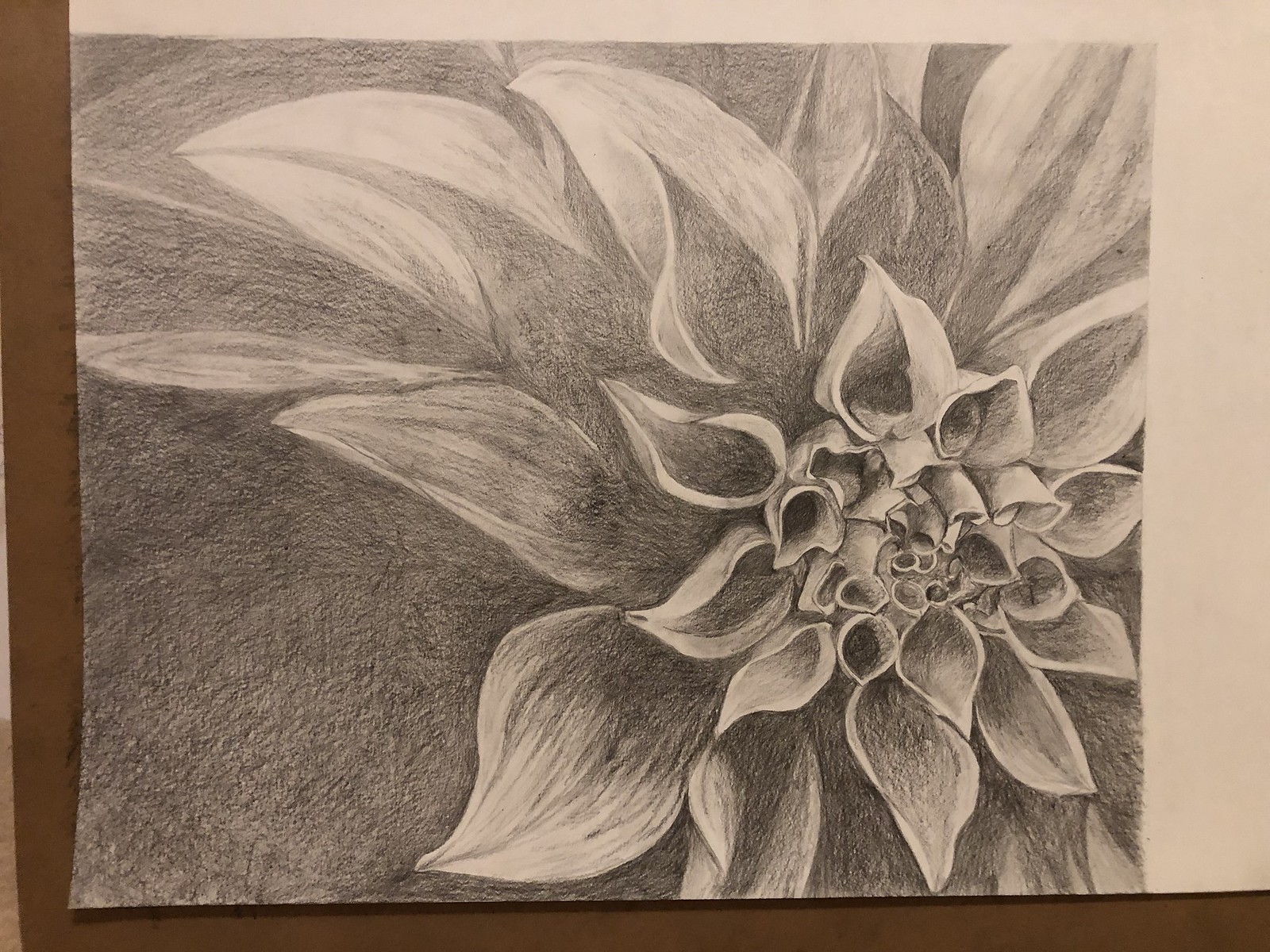A finely detailed drawing of a flower, rendered in charcoals and pencil, rests on light sepia-toned, off-white paper, placed against a brown surface. The flower's petals transition from large, open leaves on the outer edges to smaller, tightly closed buds as they approach the center, creating a compelling sense of depth and dimension. The intricate shading, ranging from deep blacks to gentle grays, vividly enhances each petal's texture and contours, making the individual strokes of the artist's hand visible. The surrounding background is etched dark, framing the flower and adding emphasis to its delicate structure. Despite the monochromatic palette, the shading's complexity invokes a sense of imagined color, enriching the visual experience. The flower's center is positioned about three-quarters of the way across the page, surrounded by approximately thirty petals that display varying levels of openness, all depicted with exceptional detail and care. The image is both striking and serene, beautifully capturing the essence of nature through the art of sketching.